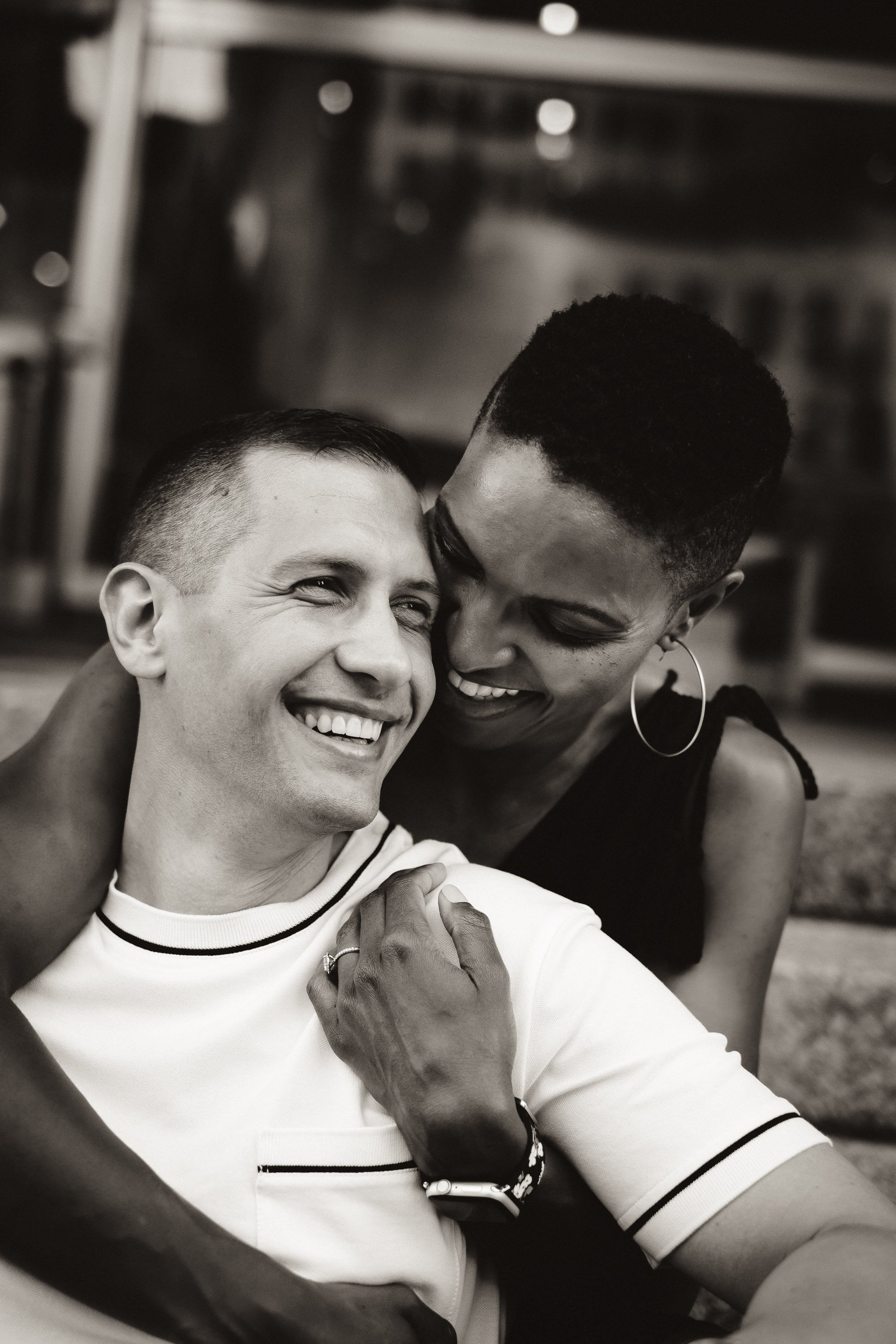In this black-and-white photograph, a loving couple is captured in an affectionate embrace. The man, who has light skin and an Eastern European appearance, is positioned in the foreground. He has a broad smile on his face and is wearing a white t-shirt adorned with black stripes around the pocket, arm, and neckband. His arms rest casually by his sides. Behind him, the woman with darker skin and short black cropped hair leans her cheek against his, her head tilted slightly downward. She is smiling warmly, her arms wrapped around his chest and shoulder, lightly gripping his shoulder with her fingers. She is dressed in a black sleeveless shirt, large silver hoop earrings, and a silver wristwatch on her left arm. The background is blurred, suggesting they might be near a building with a light shining above, though the focus remains solely on their tender moment. This intimate scene beautifully captures the love and connection between the interracial couple.